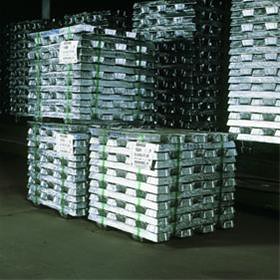In this photograph taken at a shipping warehouse, multiple stacks of crates are meticulously organized on a dark gray cement floor. In the foreground, there are two crates side by side with another crate stacked on top. Behind this arrangement, a multitude of other crates are similarly stacked, all uniformly fitting together with the layers conjoining perfectly. Green wires, used as ties, are visible hanging from some of the crates, while inside the crates, white trays can be seen though the contents are not clearly distinguishable. On the crate in the upper left-hand corner, there's a white square sign with text that's too distant to read clearly. The overall scene is an orderly display of crates prepared for storage or future use.